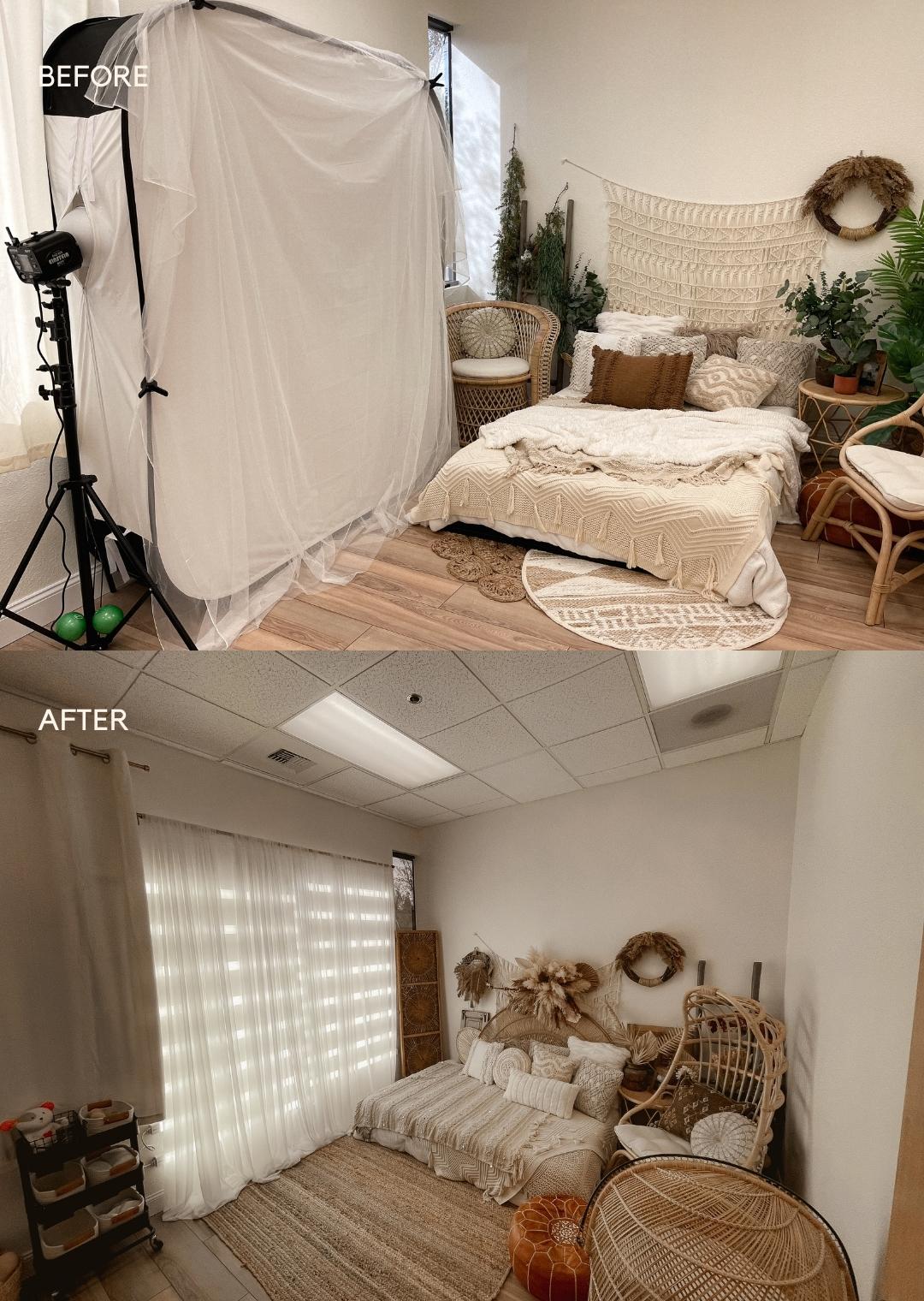The image depicts a dramatic transformation of a bedroom through a before and after comparison. In the cluttered "before" picture, we see a bedroom filled with an abundance of greenery, including several plants, and a low bed covered with a beige textured bedspread and a furry tan blanket. The room is decorated with a woven wall hanging behind the bed, a makeshift clothing storage unit, a video camera on a tripod, and two green balls, creating a very busy atmosphere. The wooden floor has a round area rug partially covering it, and there's a wicker chair and table. The walls are white, contributing to the neutral color palette of tans and browns.

In the organized "after" picture, the bedroom has undergone a stylish makeover. The makeshift storage unit and camera equipment have been removed, allowing beautiful curtains and a window to be showcased. The bed looks much neater with a cleaner, more coordinated comforter, surrounded by several decorative pillows. A new headboard featuring dried beige plants has replaced the macrame wall hanging, adding a fresh touch. The floor no longer has a small rug but is fully carpeted instead, enhancing the unified look. A wooden shelf has taken the place of the plants, and a comfortable wicker chair remains in the corner, complemented by new, intricate rattan furniture. The overall aesthetic is still natural and neutral, but far more orderly and visually appealing.